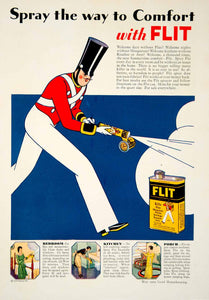This vintage vertical advertisement, likely from the 1920s and styled in an Art Deco font, promotes FLIT, a household spray product. Central to the ad is a cartoon figure resembling a toy soldier or drummer boy, dressed in a red long-sleeve coat with criss-crossing white sashes, white buttons, white pants, and black boots with yellow soles. His tall black hat with a chin strap and black-and-yellow cuffs add to his old-timey appearance. He is depicted holding a spraying device, emitting a large cloud of FLIT, echoing the tagline "Spray the way to comfort with FLIT" in bold capital letters. The advertisement's yellow and black rectangular FLIT can is prominently displayed beneath the cloud. At the bottom, three illustrations show women using FLIT in various domestic scenarios, emphasizing its everyday utility. The blue and white background further accentuates the ad's vintage charm.